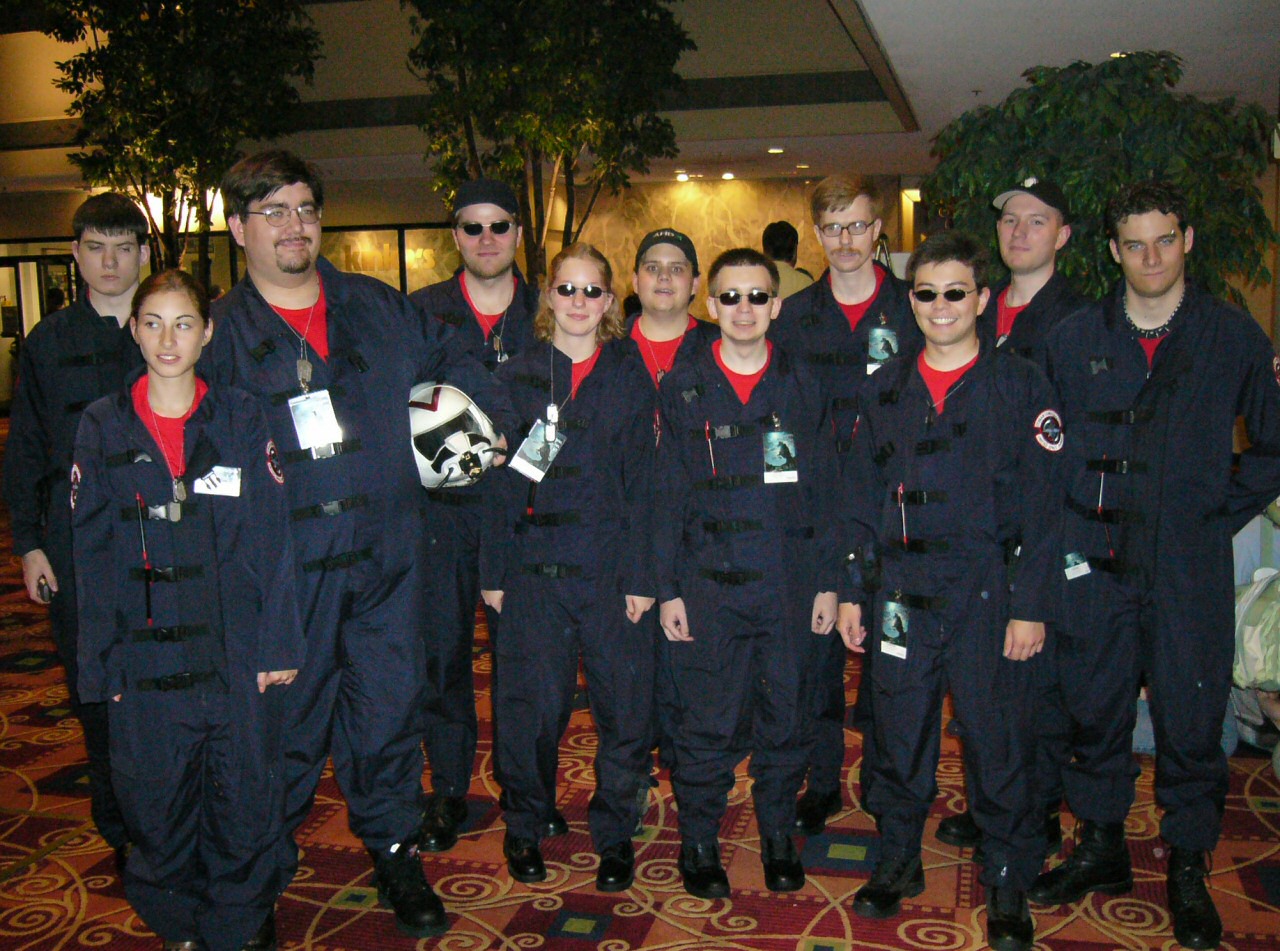The photograph captures a group of people standing shoulder-to-shoulder, each dressed in dark blue one-piece suits that resemble flight suits. Underneath these suits, they wear red shirts, and they all sport uniform black leather shoes or shiny black boots. One of the individuals, positioned towards the back, holds a helmet. The group is composed of men and women ranging in age from their early 20s to middle-aged, with a predominant majority appearing Caucasian, although there's a single Asian male on the far right. Most participants have light skin tones. Several of them are wearing sunglasses, adding to a uniform appearance.

They stand in what appears to be a hotel lobby, characterized by an orange carpet with darker orange and yellow swirl designs. The backdrop features a gold wall, a white ceiling, potted indoor plants, and sliding glass doors visible on the left side of the image. Notably, the setting includes what seem to be artificial trees spaced around the group. Despite the lack of clarity regarding their organization or reason for uniformity, the group exudes a cohesive and friendly demeanor.